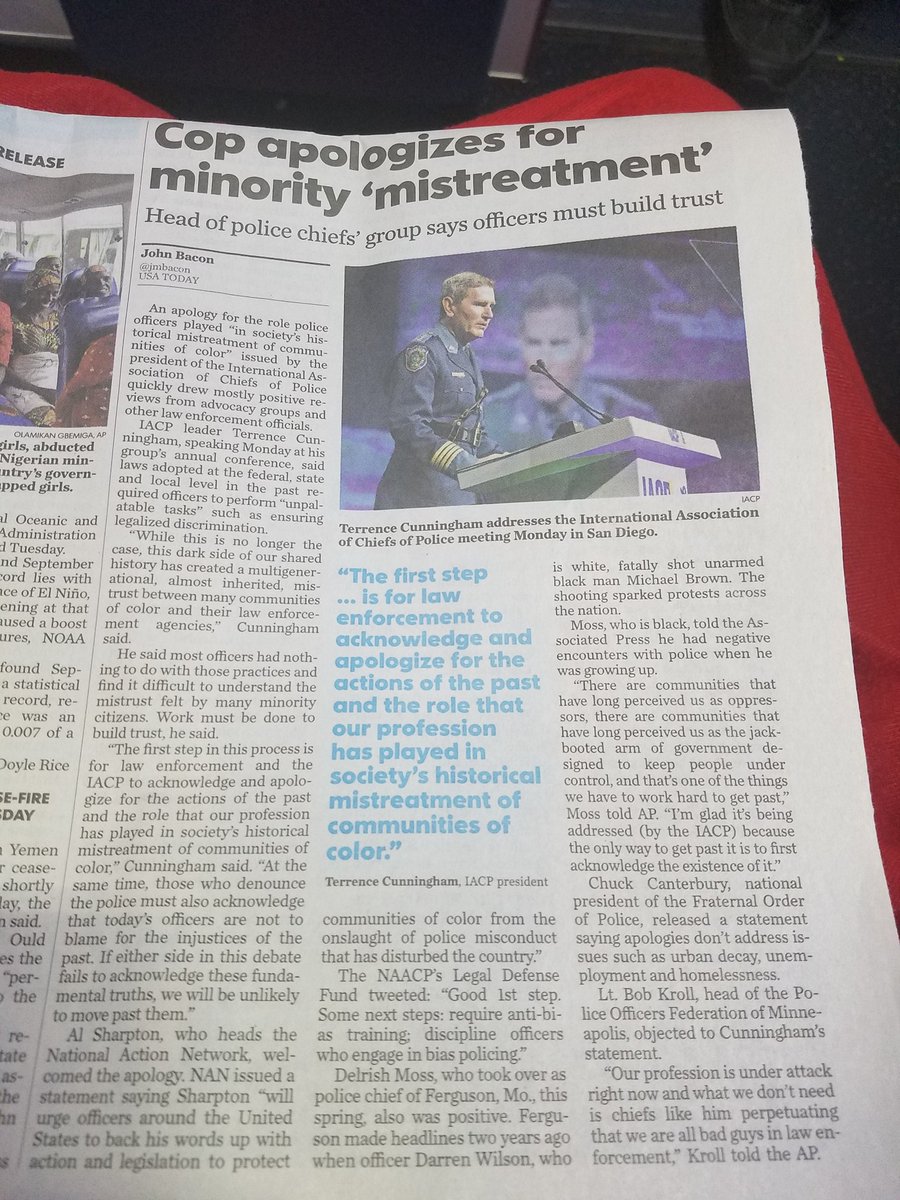In this detailed photograph, a newspaper rests on someone's lap, the person wearing vibrant red pants. The setting appears to be inside an airplane, as evidenced by the visible black and silver elements that resemble seat armrests and seat backs in front of the individual. The newspaper itself is printed on a grayish paper and prominently features a headline: "Cop Apologized for Minority Mistreatment: Head of Police Chief Group Says Officers Must Build Trust" by John Bacon from U.S. Today.

The news article captures a significant moment where the president of the International Association of Chiefs of Police (IACP), Terrence Cunningham, publicly apologized for the historical mistreatment of communities of color by the police. Speaking at the IACP's annual conference, Cunningham acknowledged that federal, state, and local laws once mandated officers to enforce discriminatory practices, contributing to deep-seated mistrust and strain between law enforcement and minority communities. Advocacy groups and fellow law enforcement officials largely received Cunningham's apology positively, noting it as a crucial step toward rebuilding trust.